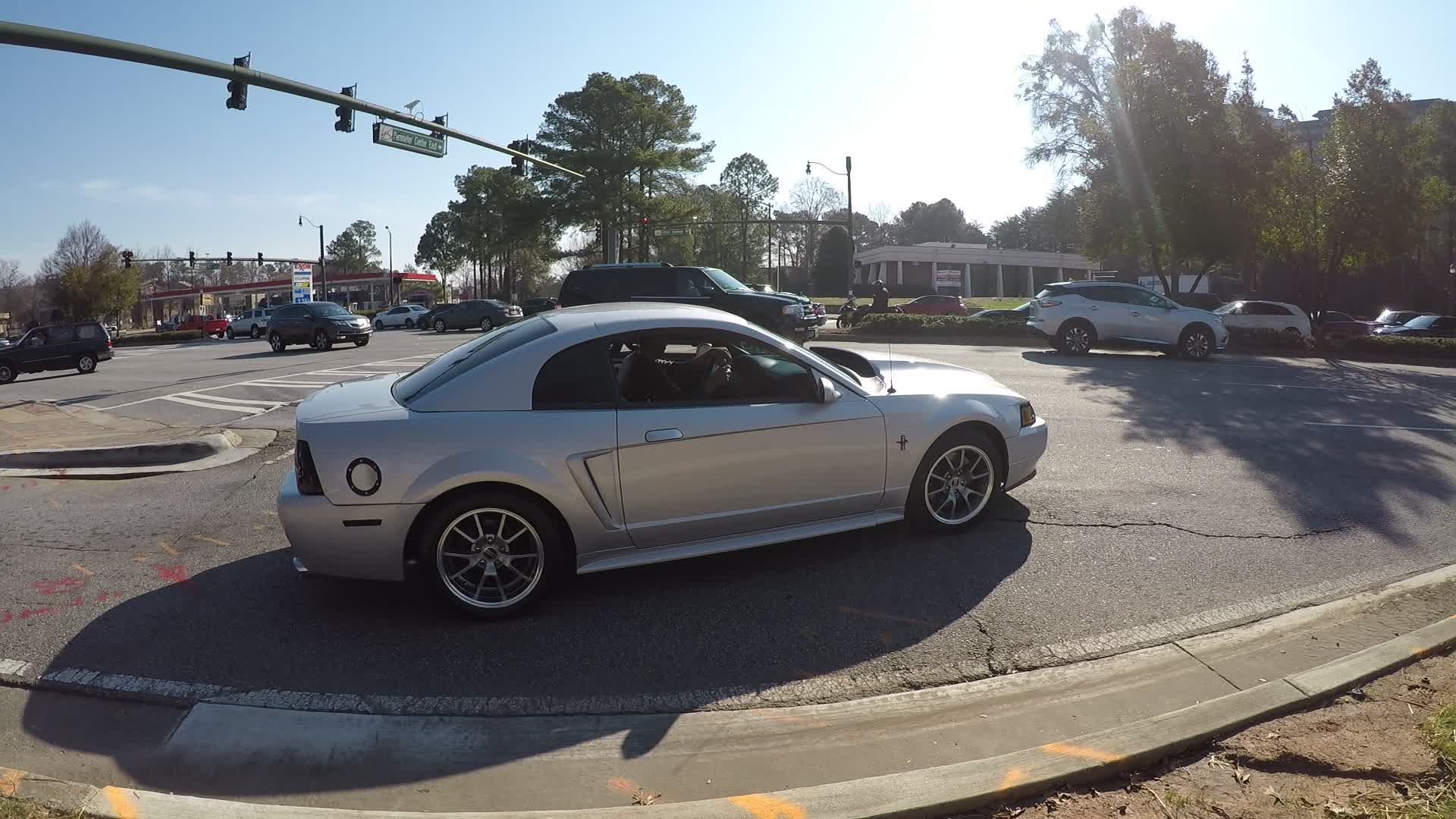This is a detailed, color photograph taken during daytime in an urban setting, depicting a street scene with a turning lane and various elements in the background. Central to the image is a shiny, bright gray compact car with a driver inside, captured from a side view as it exits the turning lane, yielding to other vehicles. The car is positioned along a sidewalk with a drain. Surrounding the scene are multiple vehicles, both parked and in motion. To the left, there is a gas station with a red roof, possibly an Exxon, featuring a red pickup truck and a silver SUV. On the right side, a parking lot is visible, filled with cars, including a white compact SUV. In the distance to the right, a low-lying light-colored building with large, dark windows is partially obscured by green, tall trees, likely palm trees indicating a location such as Florida. Above, street lights extend over the road, and the sky is a clear, sunny blue.